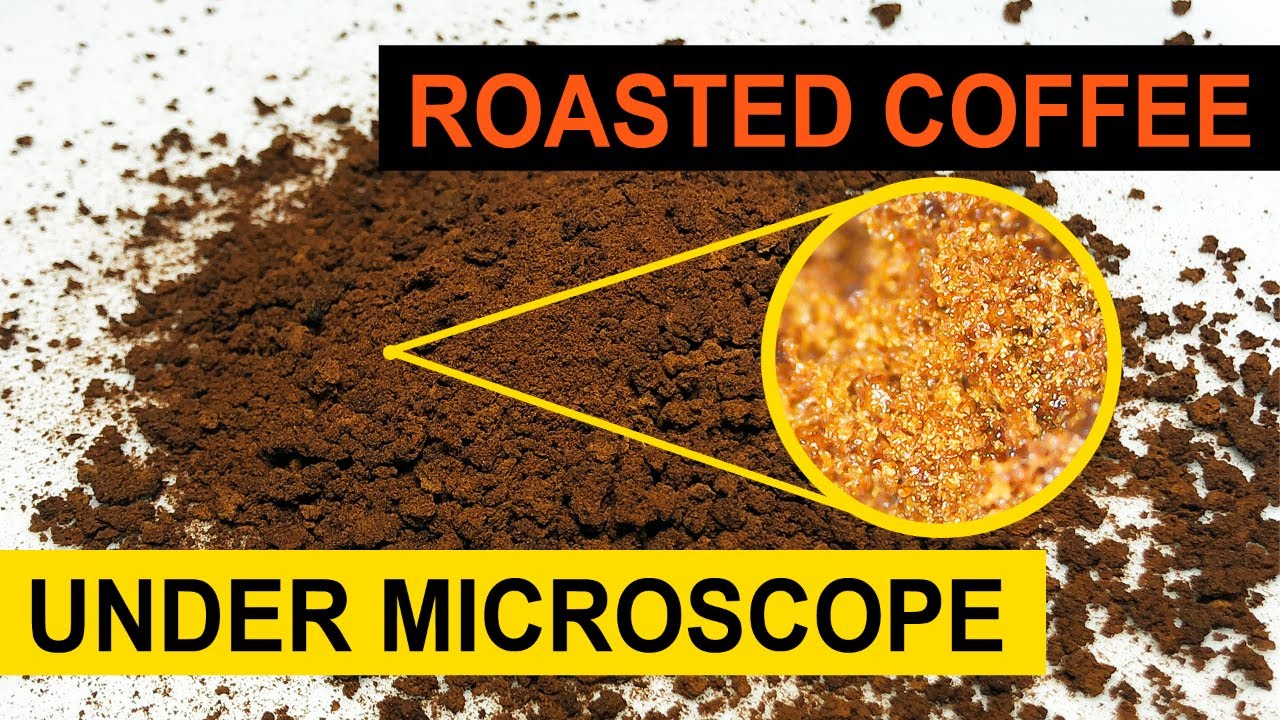The photograph features a white table scattered with dark brown roasted coffee grounds. At the top, a black banner with orange capital letters announces "ROASTED COFFEE." Below, a yellow banner with black capital letters reads "UNDER MICROSCOPE." The centerpiece of the image is a detailed yellow circle with arrows pointing inwards, highlighting a close-up view of what coffee looks like under a microscope. This microscopic view reveals clusters of coffee that appear golden and almost crystallized, starkly contrasting with the dark brown coffee grounds on the table. The image combines visual elements to emphasize the scientific examination of roasted coffee.